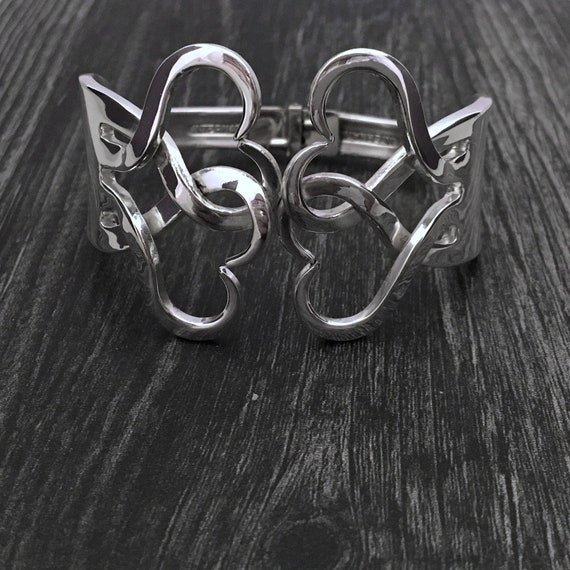The image features a shiny silver bracelet resting on a black wooden surface, which could be either a table or a dresser. The bracelet is an intricate design of two interwoven hearts on both the front and back. These hearts, with rounded tops, form little hooks that allow the bracelet to open and close without the need for a clasp or chain. Measuring approximately two to three inches wide, the bracelet emits a reflective, polished finish. The heavy-duty metal craftsmanship and heart motif give the piece an elegant and interconnected appearance.